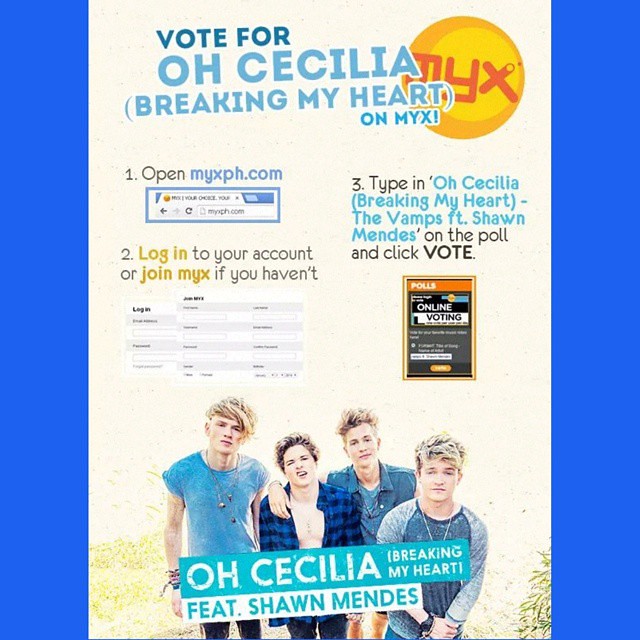The flyer, likely created by the band, promotes voting for the song "Oh Cecilia (Breaking My Heart)" on MYX. The poster features a white background with blue fonts and a bright, navy blue border. At the top, it reads "Vote for 'Oh Cecilia (Breaking My Heart)' on MYX," indicating the title of the song by The Vamps featuring Shawn Mendes. Below the title, it provides clear instructions for voting: 

1. Open myxph.com.
2. Log in to your account or join MYX if you haven't.
3. Type in "Oh Cecilia (Breaking My Heart)" by The Vamps featuring Shawn Mendes in the poll section and click vote.

Beneath the instructions, there's an image depicting the band facing the front, along with the text "Oh Cecilia (Breaking My Heart) featuring Shawn Mendes" above them. The overall design is modern yet simple, with minimalistic graphics, suggesting it might be an early promotional piece for Shawn Mendes or self-funded by the band. The poster aims to encourage online voting through MYX's portal by visually presenting the step-by-step process alongside a photograph of the band members.